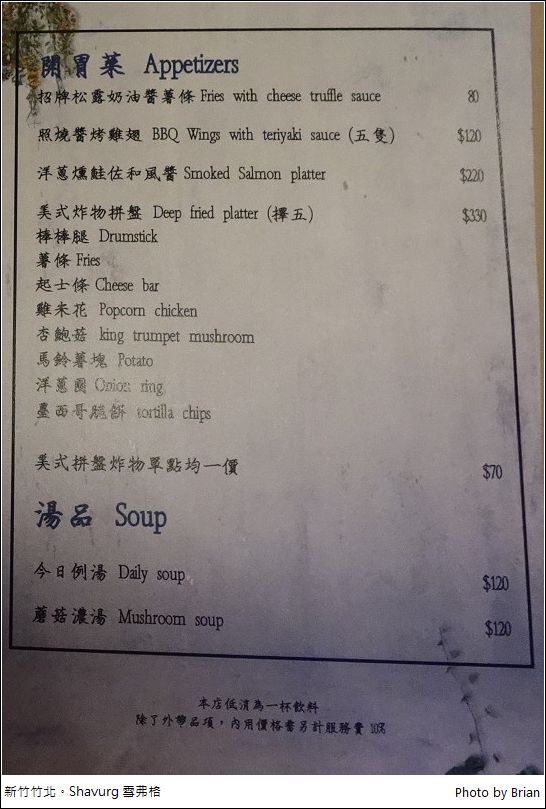A photograph captures a stained paper menu, possibly from ink bleed. The menu's background is white with a blue border, featuring a mix of Chinese characters and English translations. At the top, "Appetizers" is indicated alongside three Chinese characters. The menu lists:

1. Fries with cheese truffle sauce - 80 (likely Hong Kong dollars)
2. BBQ wings with teriyaki sauce (followed by two Chinese characters, price unclear)
3. Smoked salmon platter - 220 or 200 (price is partially obscured)
4. Deep-fried platter (followed by Chinese characters) - priced at 330 or unreadable

Subsequent items include Chinese characters leading English translations without prices:
- Drumstick
- Fries
- Chinese bar
- Popcorn chicken
- King trumpet mushroom
- Potato
- Chicken ring or Chinese ring 
- Tortilla chips

A completely untranslated item of Chinese characters is priced at 70.

The "Soup" section lists:
- Daily soup - 120
- Mushroom soup - 120

The menu concludes with two lines of Chinese text at the bottom.

Framing the entire image, there's a thin black border with a white band along the bottom, inscribed with Chinese characters and the word "Shavurg," followed by more characters. In the bottom right corner of this band, it states "Photo by Brian." The top right of the photo shows a slim wedge of the table beneath the menu, suggesting the menu's placement. Vegetation or illustrations decorate the bottom right and top left corners of the menu.